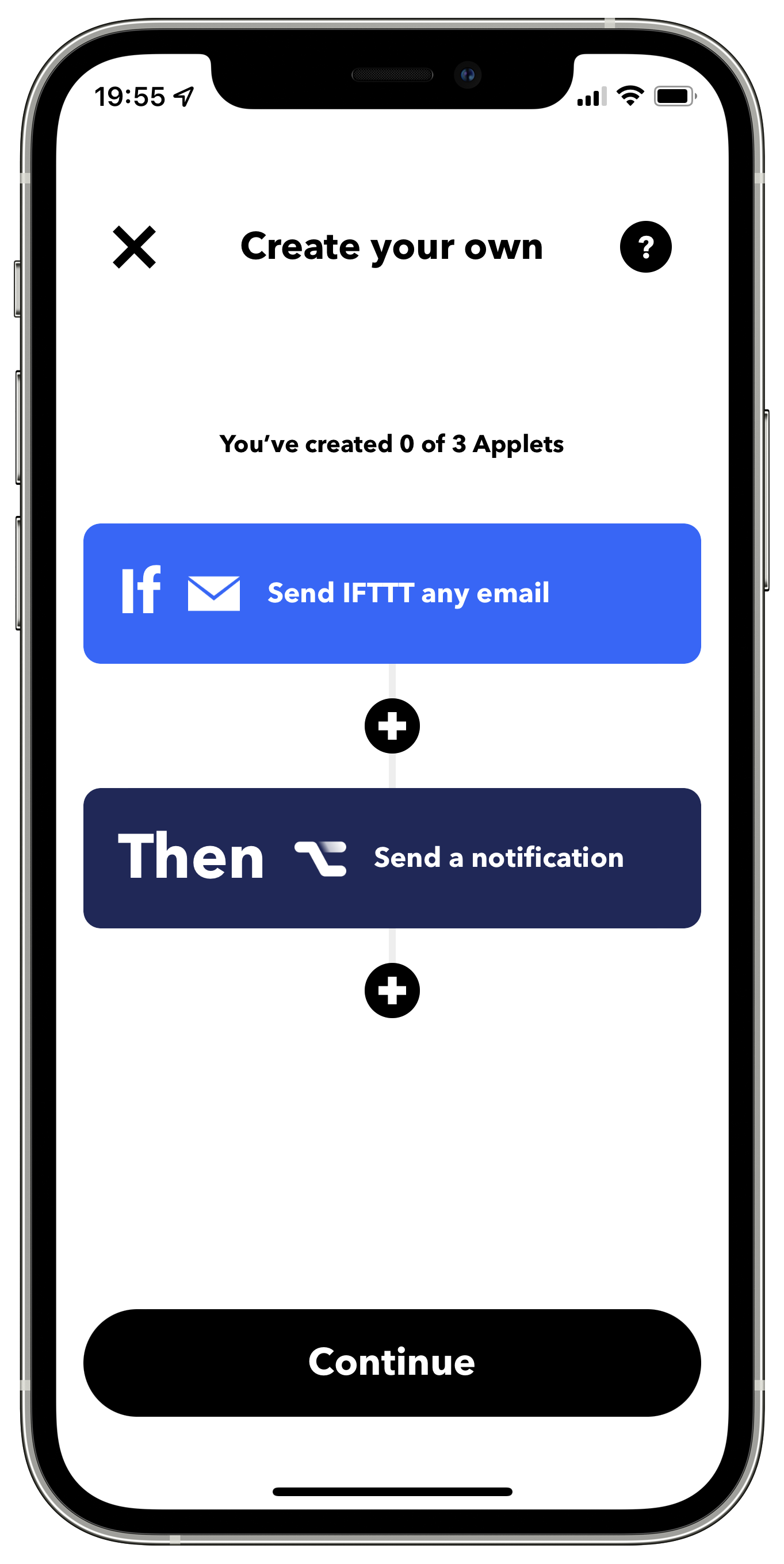The image depicts an iPhone, showcasing the device's bezel, including the volume buttons and silent switch on the left side, and the screen on/off power button on the right side. 

The phone features a prominent notch at the top, housing the clock display on the left and icons for battery level, cellular reception, and Wi-Fi status on the right. The iPhone screen displays a predominantly white background with black text stating "Create your own," accompanied by a black "X," a question mark, and a black circle to the right.

Below this, the text indicates, "You've created 0 of 3 applets," followed by a blue button labeled "if" featuring an envelope icon and the text "Send IFTTT an email." Beneath this button is a black plus icon with a white plus symbol.

Further down, a black button with white text reads "then send a notification," followed by another white plus icon on a black background. The interface also includes some white space, leading down to a black "Continue" button with white text at the bottom. 

The iPhone's universal home bar is visible at the bottom of the screen, set against the device's bezel. This comprehensive layout effectively demonstrates the phone's physical features in conjunction with a specific app's user interface.